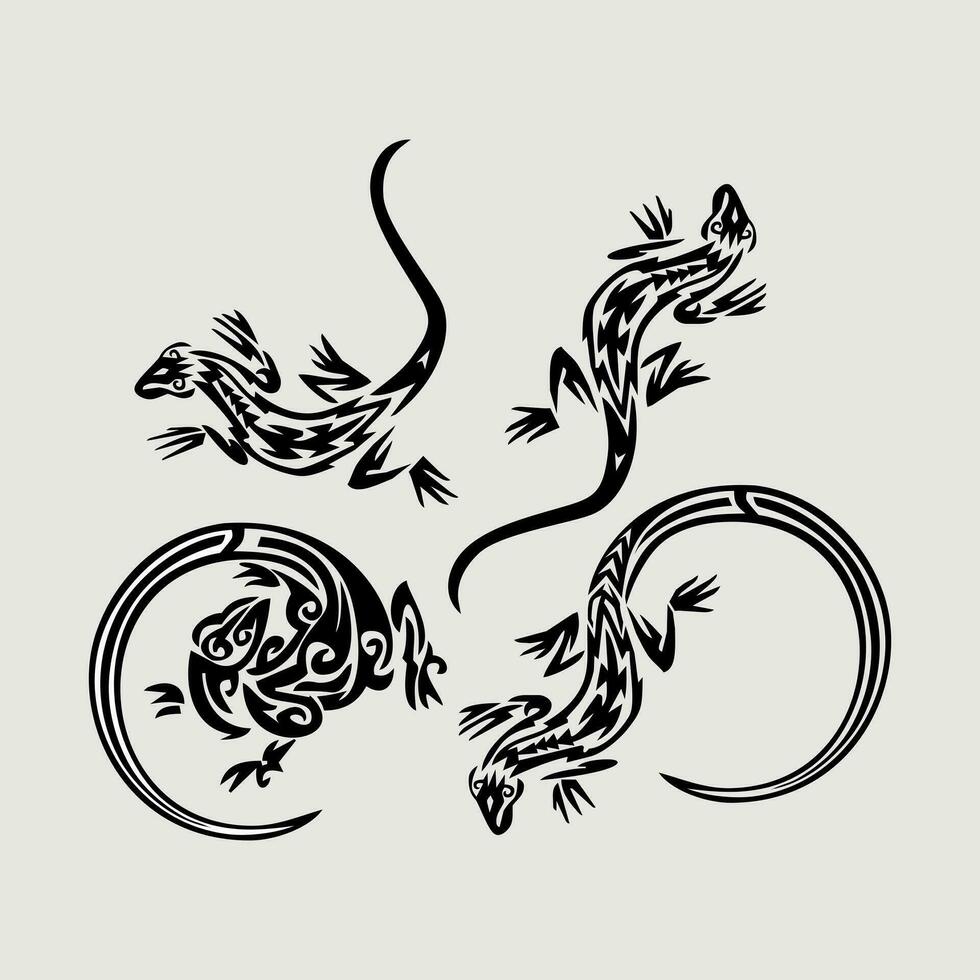The image features a photograph of a detailed drawing set against a light, soft grey or cream background. The main focus is on four stylized lizards, which appear as tattoo designs with tribal aesthetics. Each lizard has distinct features, such as long black tails and four feet, creating fluid shapes. The tails and bodies form varying shapes: one tail loops to form a circular or 'C' shape, another looks as if it’s climbing, one seems to be slithering, and another has a wavy, undulating body. These lizards are depicted in a manner that might evoke the image of a bicycle, with the looping tails resembling wheels. The intricate, black linework contrasts sharply against the subdued background, highlighting the unique and artistic quality of these designs.